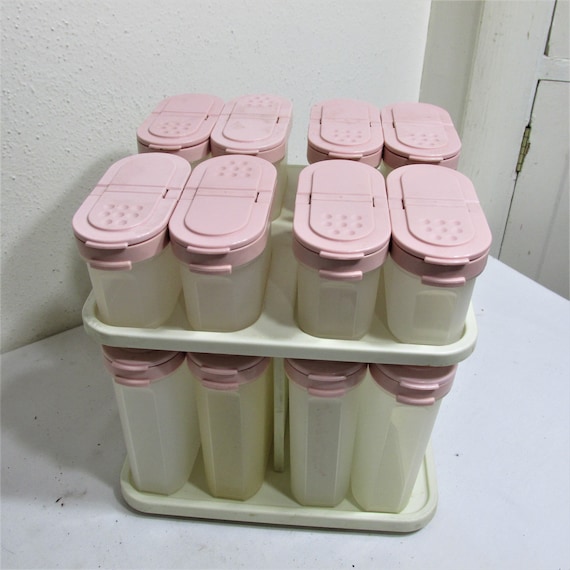This photograph features a neatly arranged display of sixteen cylindrical prism-shaped containers, organized on a two-tier white plastic shelf. Each tier holds eight containers, resulting in a total of eight on the top shelf and eight on the bottom one. The containers themselves are clear with a pale pink, dual-opening lid that allows either the entire top or just a portion to be opened. These containers are designed to stack neatly within their designated slots on the shelf.

The setup sits on a white table, which appears somewhat dirty, and serves as the central focus of the image. The background showcases a white wall with a popcorn texture and glimpses of faded white cabinets with metal hinges. The right top corner of the picture reveals part of a door hinge, emphasizing the domestic setting. The precise and organized arrangement, coupled with the pristine presentation of the containers, suggests an intentional and well-maintained storage solution.